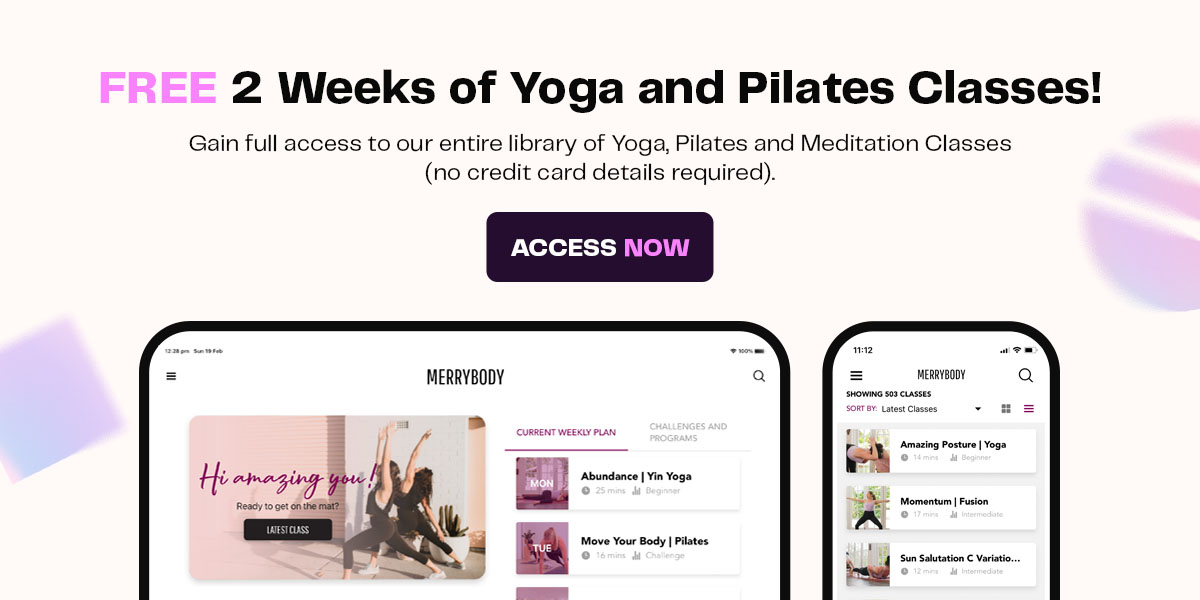This is an advertisement likely sourced from social media or a website, featuring a pale cream background. On the left side of the advert, a square shape is depicted, while the right side showcases a circle intersected by two lines. Both shapes gracefully transition through shades of blue, mauve, and pink.

At the top of the advertisement, a headline boldly announces, "Free Two Weeks of Yoga and Pilates Classes." The word "Free" stands out in bright pink, contrasting with the black text of the remaining sentence. Directly underneath, a subscript in black font proclaims, "Gain full access to our entire library of Yoga, Pilates, and Meditation classes," with an additional reassuring note in parentheses: "(No credit card details required)."

Centrally positioned within the advert is a prominent black button labeled "Access Now," where "Access" is written in white, and "Now" is highlighted in the same vibrant pink as the word "Free."

Beneath this button the advert displays images representing website and mobile interfaces. The first image possibly shows a computer or laptop screen, though the presence of the date and time in the top right corner suggests it could depict an iPad. Centrally, this screen displays "Merry Body," presumably the name associated with the advertisement. A large image of two women performing yoga is featured, with the motivational phrase "You High Amazing" in pink overlaying it. To the right, thumbnails present various yoga classes and their details.

On the right side of the advert, an outline of a cell phone screen is shown. This screen also features the "Merry Body" branding at the top, followed by thumbnails that link to different exercises and their corresponding descriptions.